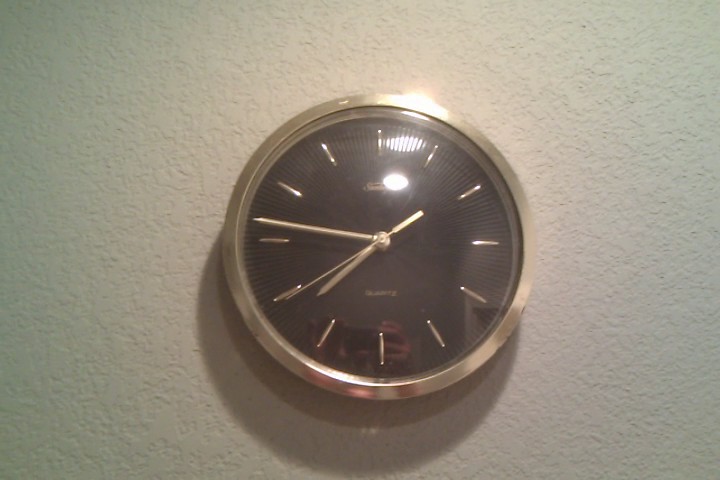The image depicts an indoor scene with a prominently featured clock mounted on a wall. The wall background appears textured and is a cream or beige color, though it has a brighter, almost white appearance due to light reflection. The clock itself is small, round, and the central focus of the picture. It is encased in a shiny gold bezel and has a black face. The clock's indicators, including the hour, minute, and second hands, are all a yellow gold color. The hour and minute hands are thicker, whereas the second hand is thinner. The time displayed on the clock is approximately 7:46 or 7:47, with the second hand near the 39-second mark.

The clock lacks numerical indicators and instead features large golden lines marking each hour. At the bottom of the clock, just above the 6 o'clock position, the word "quartz" is visible in silver, although this detail may not be easily readable. Similarly, there is additional text beneath the 12 o'clock position that is obscured by the light. The light source creates noticeable shadows below and to the left of the clock, adding depth to the image.